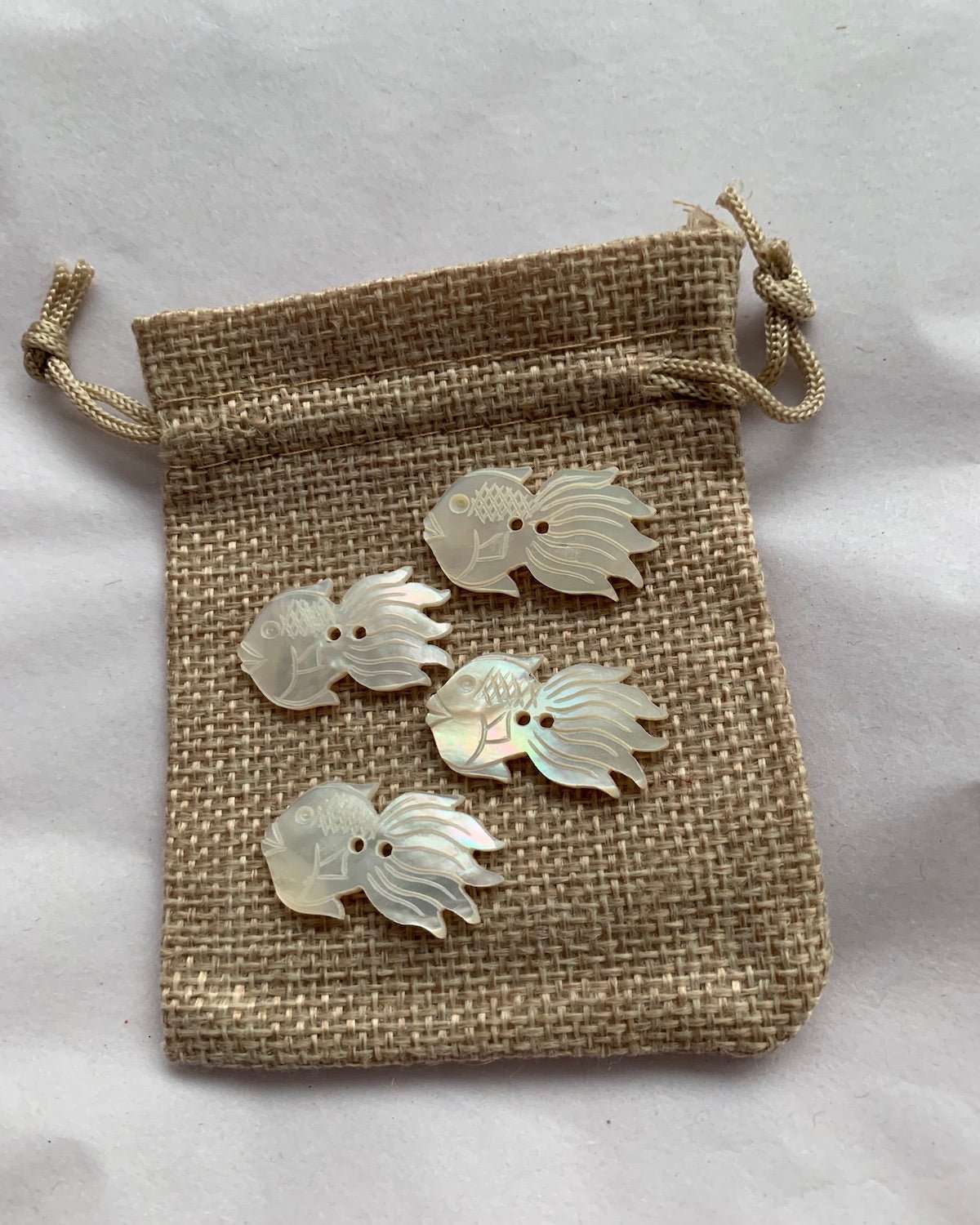The photograph showcases a small, light brown burlap drawstring bag, flattened and placed on a white, slightly wrinkled paper background. The drawstring, made of a matching cord, is untied and laid on either side of the bag. On top of the bag are four iridescent, opal-like buttons in the shape of fish, each intricately detailed with carved eyes and fins. These buttons, displaying a pearly, somewhat rainbow-shimmering finish, are not attached to the bag but are arranged thoughtfully across its surface, with their two holes visibly unthreaded.